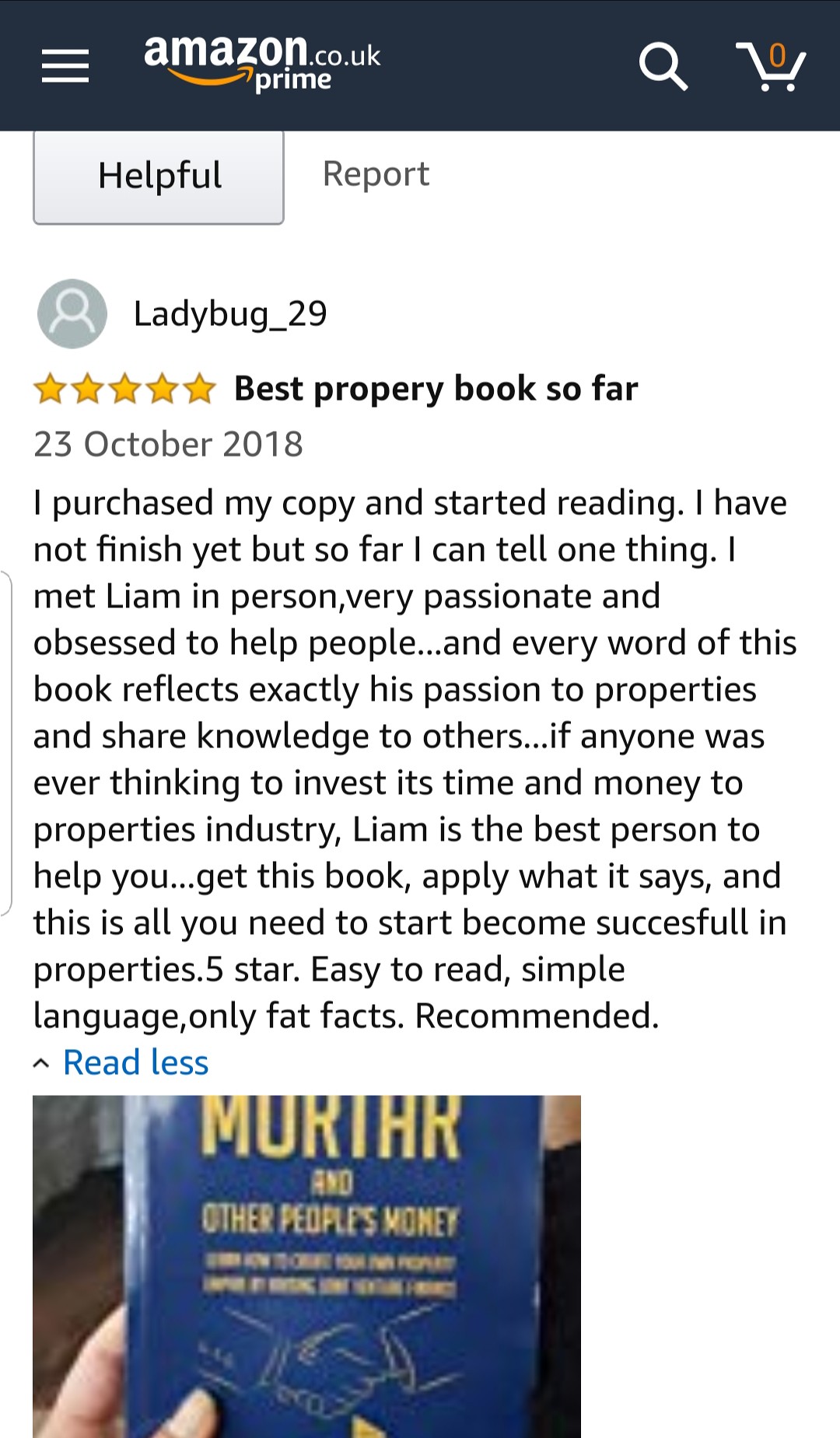This is a screenshot of a review for a property investment book on Amazon.co.uk, dated 23rd October 2018. At the top, there is a banner with white text reading "amazon.co.uk prime". The reviewer, identified as "ladybug_29", has awarded the book five out of five stars and titled their review "Best Property Book So Far." 

The review text begins in black, reading: "I purchased my copy and started reading. I have not finished yet, but so far I can tell one thing. I met Liam in person; very passionate and obsessed to help people. Every word of this book reflects exactly his passion for property and sharing knowledge with others. If anyone is ever thinking of investing time and money in the property industry, Liam is the best person to help you. Get this book, apply what it says, and this is all you need to start and become successful in property. Easy to read, simple language, only facts. Highly recommended."

Below the review, there is blue text reading "Read Less," and an image showing someone holding a blue book. The book's cover is partially visible, with the title "Mortar and Other People's Money" and a yellow outline of two hands shaking.